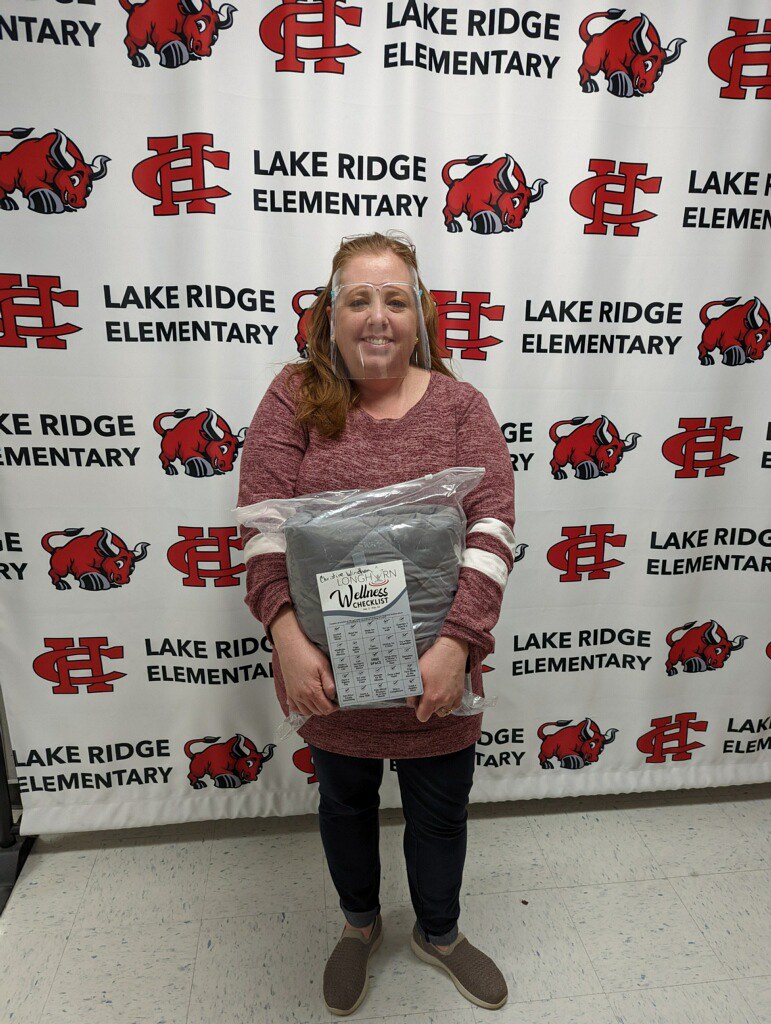In this image taken at an elementary school, a woman stands on a speckled white tile floor, posed in front of a backdrop that repeatedly displays the name "Lake Ridge Elementary" along with an associated logo featuring a red bull and intertwined letters "H" and "C." She is dressed in a light reddish, burnt red sweater adorned with two white stripes on each sleeve near the elbows, black pants, and brown slip-on shoes. The woman wears a clear plastic face mask, reminiscent of protective gear used during COVID times. In her hands, she holds a packaged gray blanket and a "Wellness Checklist" sign that prominently features the word "LONGHORN."